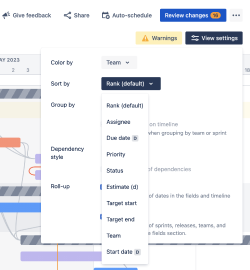This image depicts a detailed screenshot of a web application interface for project management or task tracking. The interface includes several tabs and options, such as "Give Feedback," "Share," "Schedule," and "Review Changes." There are various sections labeled "Open," "Written," "Rank," "Default," and "Rank Default." Additionally, the interface features fields for "Assign," "Due Date," "Priority," "Status," "Estimate," "Target Start," "Target End," "Team," and "Start Date," indicating a comprehensive tool for managing project timelines, task assignments, and team collaboration. The image is rich with details, suggesting a complex and robust application designed for detailed project oversight and task management.